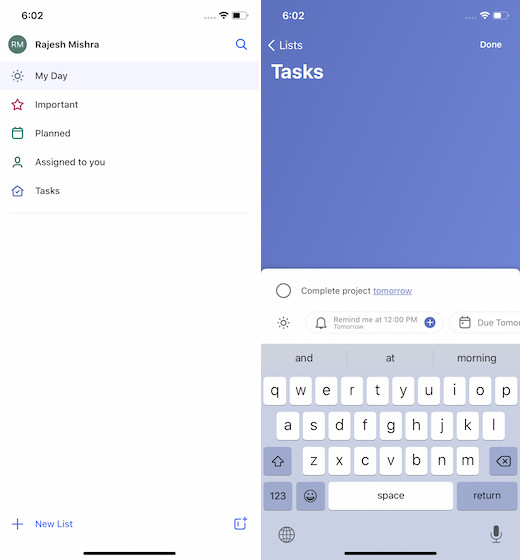A web page with a dual-window interface is displayed, showcasing a settings window on the left and an interactive section on the right, indicating it’s on a smartphone. The top left corner of the screen displays the time "6:02" without specifying AM or PM. On the top right, there are four ellipses followed by a full Wi-Fi signal icon and a battery icon showing 50% charge. Beneath this, a new section appears with a dark blue or grey circle inscribed with "RM," and the name "Rajesh Mishra" capitalized in bold black font. A dark blue magnifying glass icon is located at the far right.

Just beneath this, a highlighted grey section includes a sun icon on the left labeled "My Day" in black text. Following this, various icons are lined up each with a corresponding label: a red star with "Important," a green calendar with "Plan," a dark green person icon labeled "Assigned to you," a blue house with a checkmark labeled "Task." At the bottom, there’s a plus icon labeled "New List" and to the right, a dark blue square icon.

The right side of the interface features the same dark blue color theme and icons, alongside a QWERTY keyboard. There's an unchecked circle with "Complete project tomorrow" in hyperlinked blue text, indicating a bulleted list format.